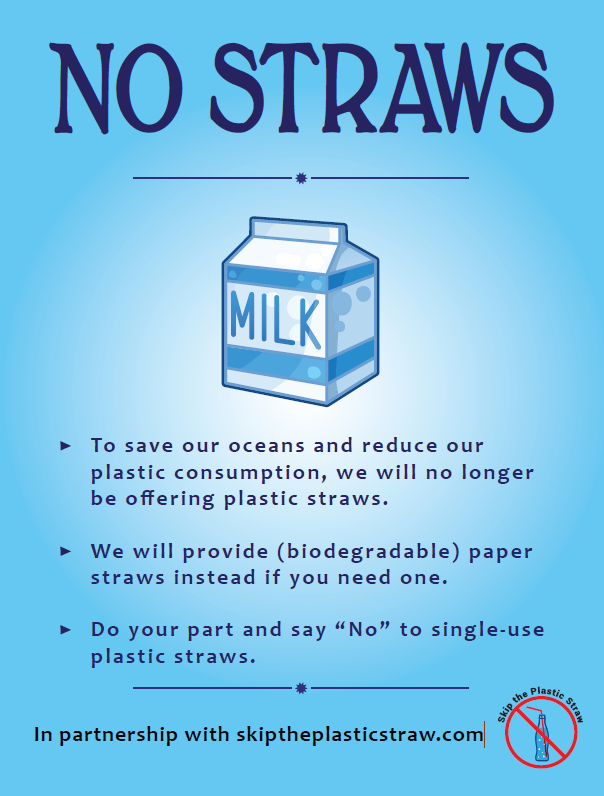This image is a portrait-oriented educational poster focusing on environmental advocacy, specifically urging viewers to avoid single-use plastic straws to protect the oceans. The background transitions from a baby blue at the edges to almost white at the center, creating a gentle gradient. 

At the top, bold, capitalized dark blue letters declare "NO STRAWS," followed by a horizontal line with a circle in the middle. Below this, a prominently featured cartoon illustration of a milk carton labeled "MILK" occupies the central upper portion of the image. This is followed by three bullet-pointed messages in descending order: 

1. "To save our oceans and reduce our plastic consumption, we will no longer be offering plastic straws."
2. "We will provide biodegradable (paper) straws instead if you need one."
3. "Do your part and say no to single-use plastic straws."

Each bullet point uses darker text for emphasis. Below these messages, another horizontal line with a circle marks the division, and at the bottom in black text, it states, "In partnership with SkipThePlasticStraw.com." 

Accompanying this text is a logo featuring a glass or plastic bottle with a straw, overlaid by a red circle and line crossing it out, symbolizing the prohibition of plastic straws. The overall color scheme includes light blue, dark blue, white, gray, and red, giving the poster a cohesive and visually appealing look, effectively conveying the public service message.